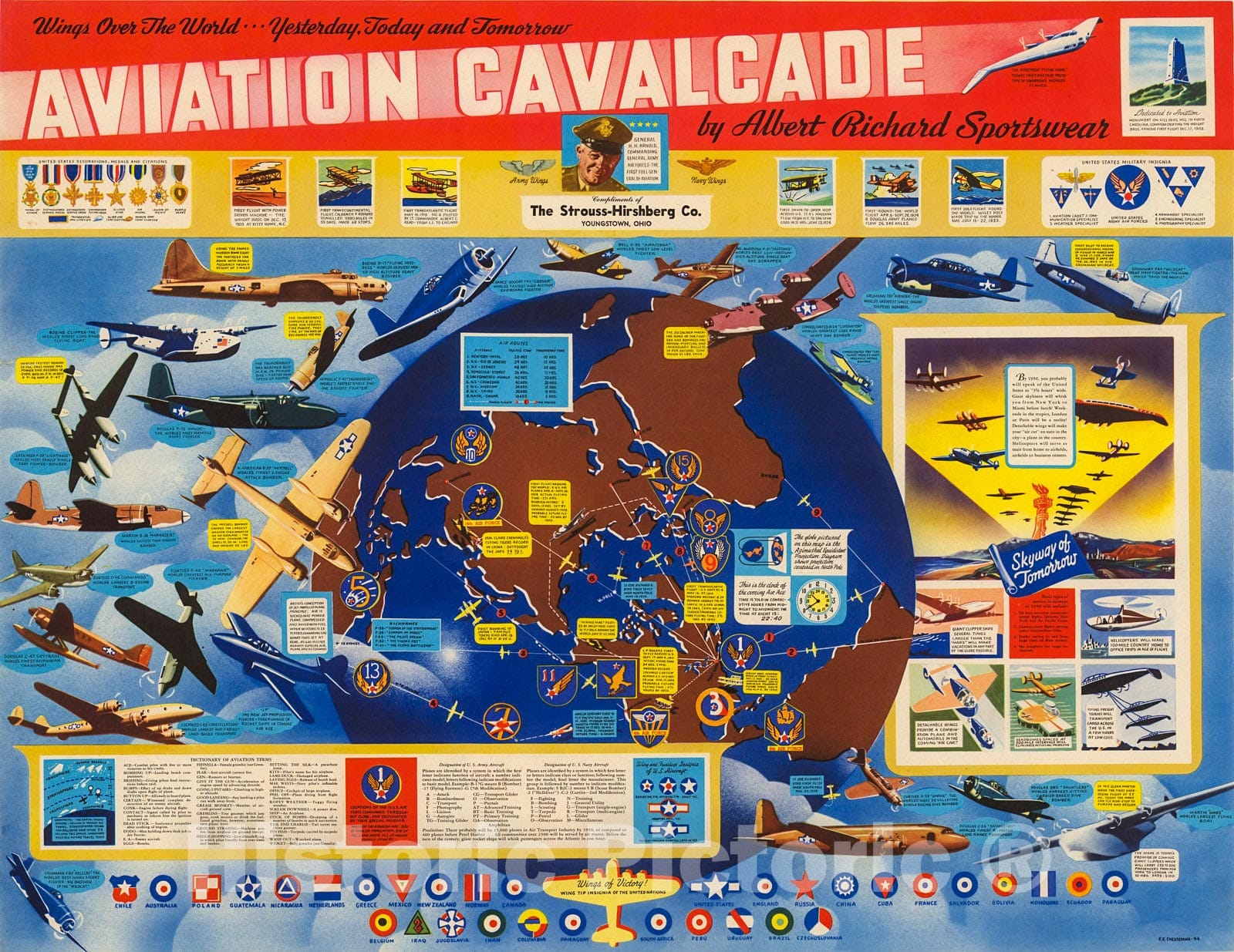The image showcases a vintage aviation poster with a prominent blue and brown globe at its center, surrounded by around 50 meticulously drawn World War II-era airplanes, each annotated with information about their manufacture or significant battles. The background is primarily blue, giving the effect of an open sky. Across the top, the title "Aviation Cavalcade by Albert Richard Sportswear" is emblazoned in red. Just above, to the left, the phrase "Wings Over the World Yesterday, Today, and Tomorrow" is written. Below the title, a yellow section features various medals on the left, while smaller airplane illustrations line the right side. In the bottom right corner, there is a rectangular inset with additional images and text about the planes. The poster also credits Straus Hirshberg Company, Youngstown, Ohio. The overall design highlights the global reach of aviation history and honors the diverse aircraft by carefully marking their origins or famous engagements with arrows and lines pointing from each plane to specific locations on the globe.